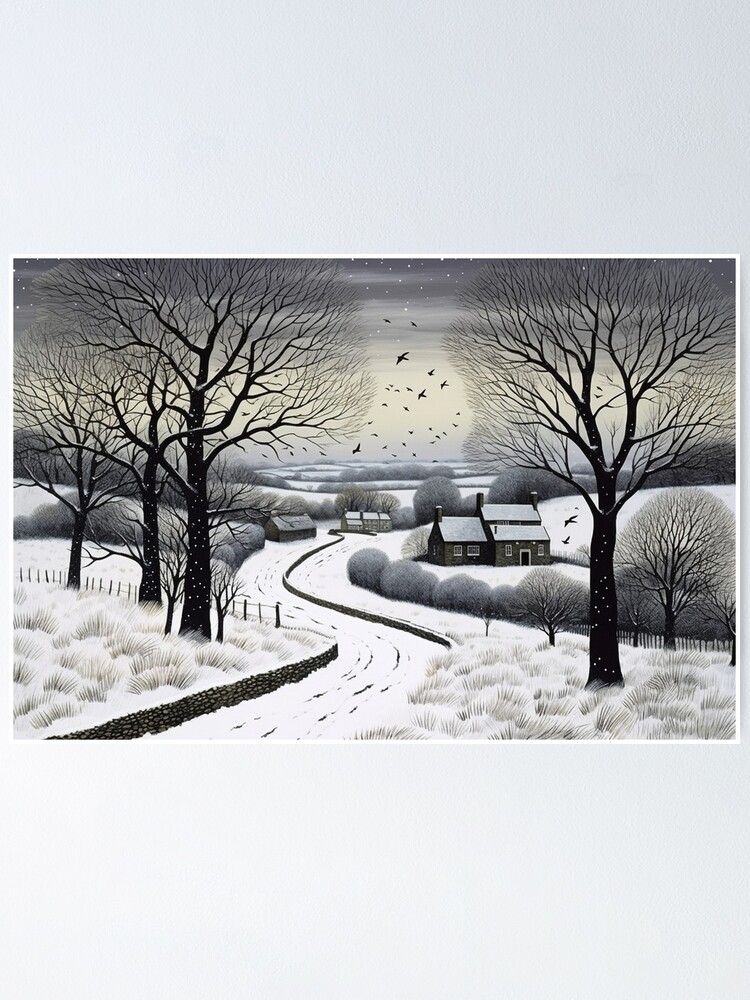The image depicts a clear, detailed wintry scene, likely a painting, set against a grey background. Dominating the center is a snow-covered path lined with grass, bushes, and large trees with dark, bare branches, evocative of a wintry forest. Smaller trees, still full, dot the snowy ground, adding contrast to the stark trunks. Flanking the path are a few homes, small and quaint, nestled into the landscape. The bright, clear sky above, tinged with a greenish dusk light and scattered clouds, is enlivened by a flock of birds in flight. The scene is well-lit and highly detailed, with no words or numbers marring the image's clarity, capturing a serene yet vibrant moment in a snowy region.